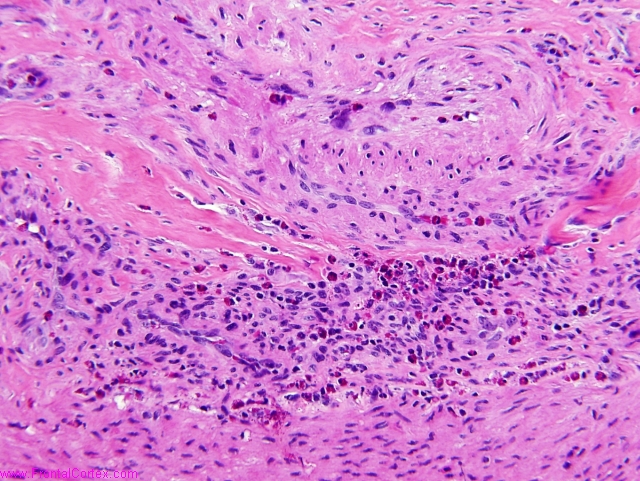This horizontal rectangular image is dominated by a predominantly pink surface featuring a complex interplay of colors and textures, reminiscent of a microscopic photograph or an abstract painting. The image is filled entirely by this design, with no other objects or text, suggesting a high magnification or a zoomed-in abstract art piece. Various shades of pink cover most of the area, accented by numerous purple dots and occasional thicker spots. Additional details include sporadic white streaks and dots distributed across the surface. In the middle of the image, there is a darker pink section resembling a river or flow, adding to the intricate pattern. Below this central flow, the purple speckles grow denser, while they appear less concentrated towards the top. The image evokes a sense of artistic style, whether it be in the realm of biological photography or abstract art suitable for display.